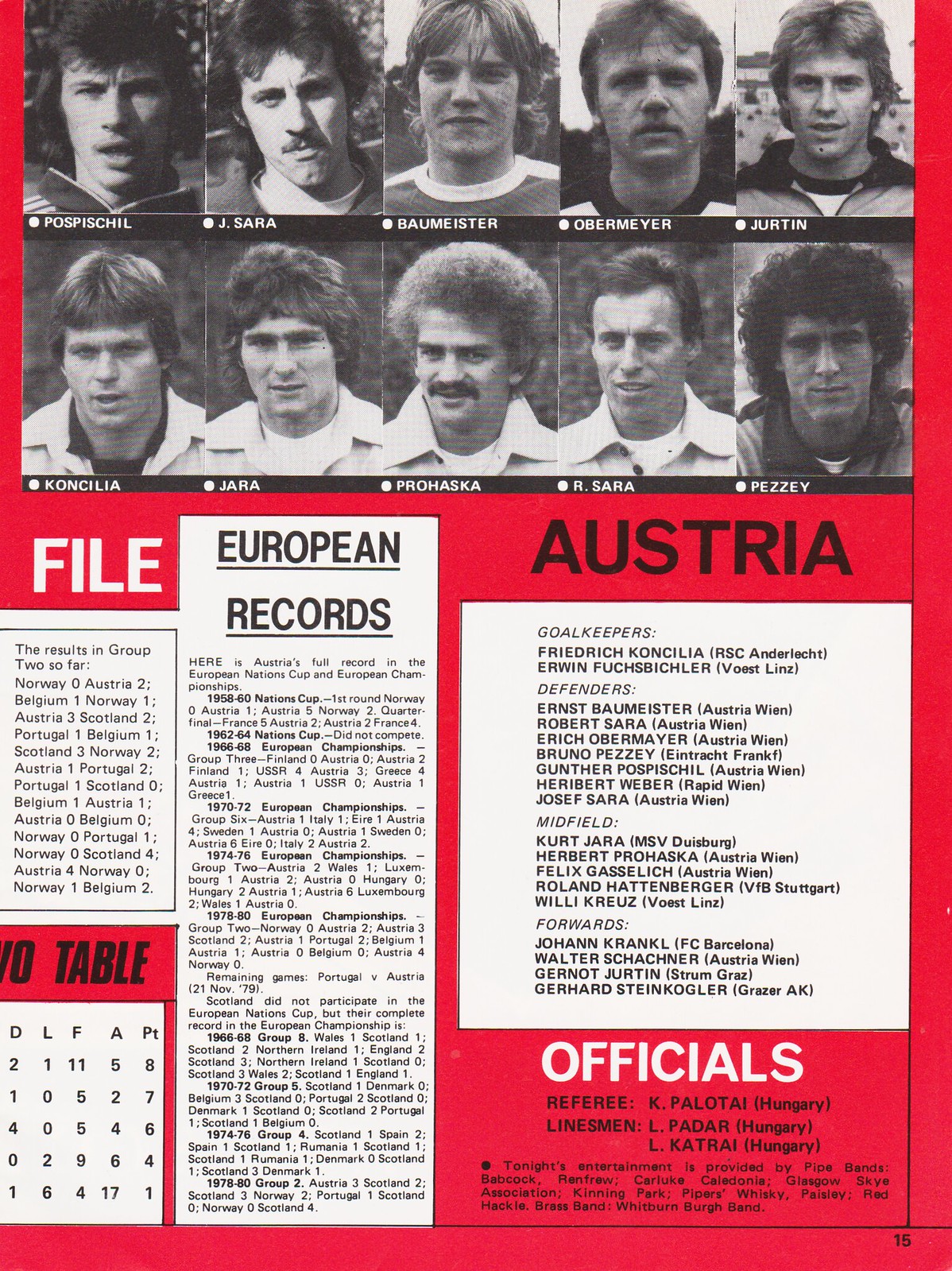The image resembles an old newspaper clipping with a solid red background. The layout is vertically aligned and presents various sections of information, predominantly related to soccer.

The top half of the image displays two rows of black-and-white photographs, each featuring five individuals, likely from the 1970s. Each portrait is labeled with the individual's last name in white letters underneath. Among the names are Popsicle, Jsara, Baumeister, Obermeyer, Jerton, Conacilia, Jara, Prochaska, Jara, Sahara, and Peasy.

Below the photographs, the section shifts to text-based content on the red background. Notably, "European Records" is prominently displayed in bold, underlined black letters. This section contains a table detailing Austria's performance in the European Nations Cup and European Championships from 1958 to 1960, listing various match results, including Austria's victories and defeats against Norway, France, Belgium, Scotland, and Portugal.

To the right, similarly styled bold black letters spell "Austria," followed by another text box listing player positions and names, including goalkeepers, defenders, midfielders, and forwards. 

At the bottom of the image, there is a section labeled "Officials" in white capital letters, listing the referee K. Pulido and linesmen L. Padar and L. Katria, all from Hungary. In the very lower right-hand corner, the number 15 indicates the page number from the original newspaper or booklet.